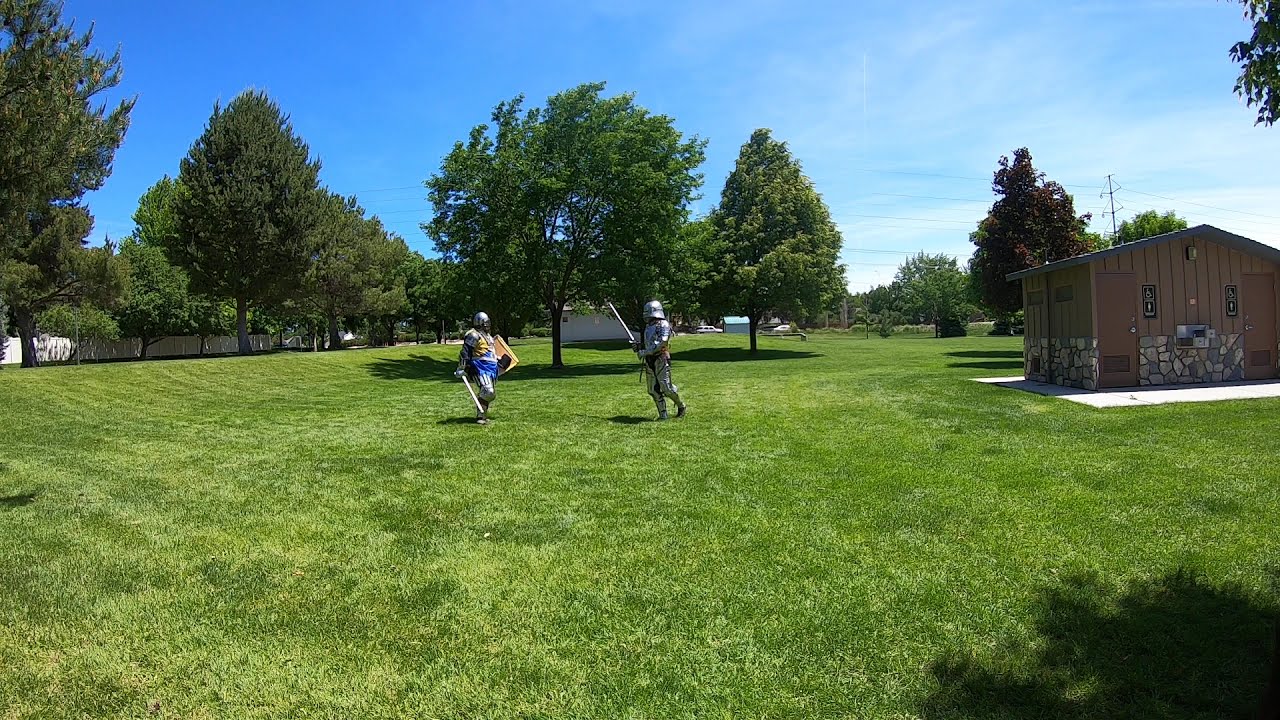In this outdoor scene, a vivid daytime sky showcases a few white clouds against an expanse of blue. The foreground is dominated by a vibrant green grass field lined with scattered trees, embodying the serenity of nature. Central to the image are two individuals dressed as knights, standing face-to-face as if preparing for a duel or re-enacting a historical battle. Their armor gleams silver under the sunlight, with metal helmets, upper body armor, and shin guards extending to their thighs. The knight on the left stands out with additional blue attire, including blue shorts over his armor, holding a sword and a shield at his side. His counterpart on the right, clad predominantly in grey and silver, has his sword raised, ready for action.

Surrounding the combatants, the background includes a small brown building with restroom facilities, noticeable by its brown doors. Further in the distance, power lines and poles interlace the scene, accompanied by a few parked cars. The photograph, taken from a standing position, captures the essence of a bright, nearly cloudless day with sunlight enhancing the various hues of yellow, blue, multiple shades of green, dark blue, teal, brown, and white that are present in the scene.